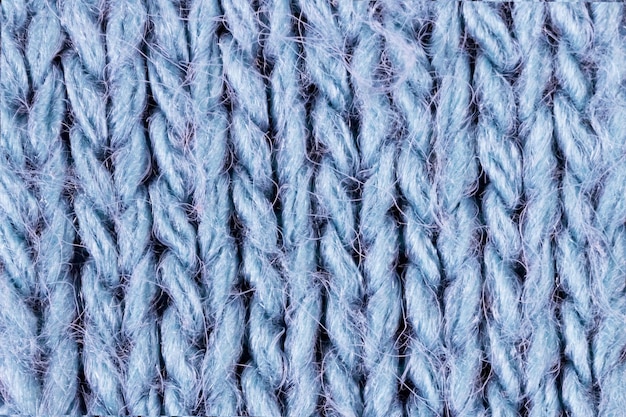This high-definition, close-up photograph captures a detailed view of what appears to be a crochet or knitted fabric. The yarn, primarily in a light ice-blue color, has stitches arranged vertically, creating a braided or chain-like pattern. The fabric consists of multiple rows, approximately eight visible threads laid out in a structured, repeating manner. Interspersed among the blue threads are fine, almost hair-like filaments in both purple and black, adding texture and detail to the composition. The image likely aims to highlight both the quality and intricacies of the yarn and the stitching technique used.